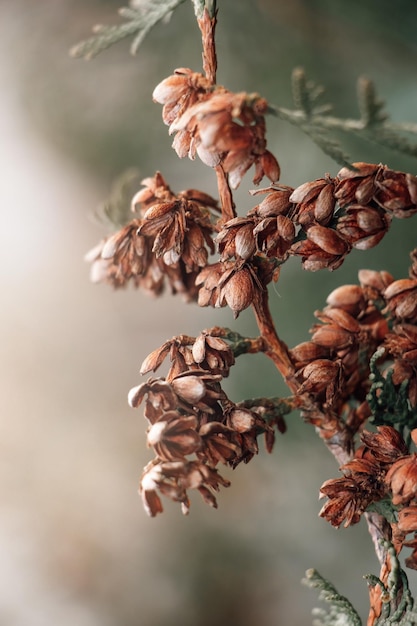This detailed photograph, taken outdoors, captures a close-up view of a lightly curved, thin tree branch, believed to be from a cedar tree, starting at the bottom right and rising diagonally before turning more vertical toward the top of the image. The branch, coated in a burnt auburn, reddish-brown hue, features clusters of almond-shaped, brown petals, resembling little pods or buds, emerging from a brown central stem. The focus is sharp on these intricately detailed elements, giving the impression of an artwork or painting. In contrast, the background is blurred, revealing vague but identifiable colors of cream, white, dark green, and brown, with a faint, blurry pine branch on the right and green needles at various points along the main branch.